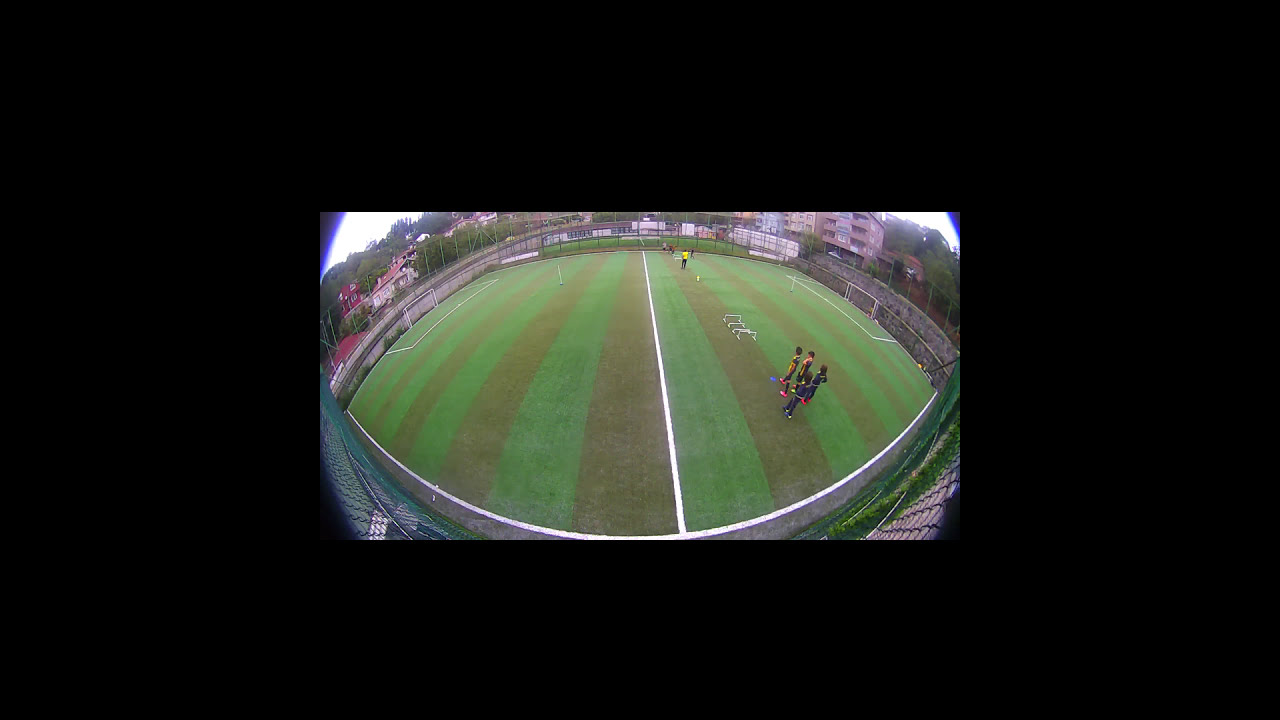The photo, taken with a fisheye lens, offers a panoramic, slightly elevated view of an outdoor soccer field. The field is well-manicured, displaying green and brown striped grass and is enclosed by a dark green chain link fence. Each end of the rectangular field features a white goal post. Toward the right side, four individuals are standing close together; two are in dark blue long sleeves and pants, while the other two wear red uniforms. Another distant figure in a white shirt with black pants stands on the same side. In the background, houses, dense trees with thick green foliage, and distant mountains are visible, adding depth to the scene.